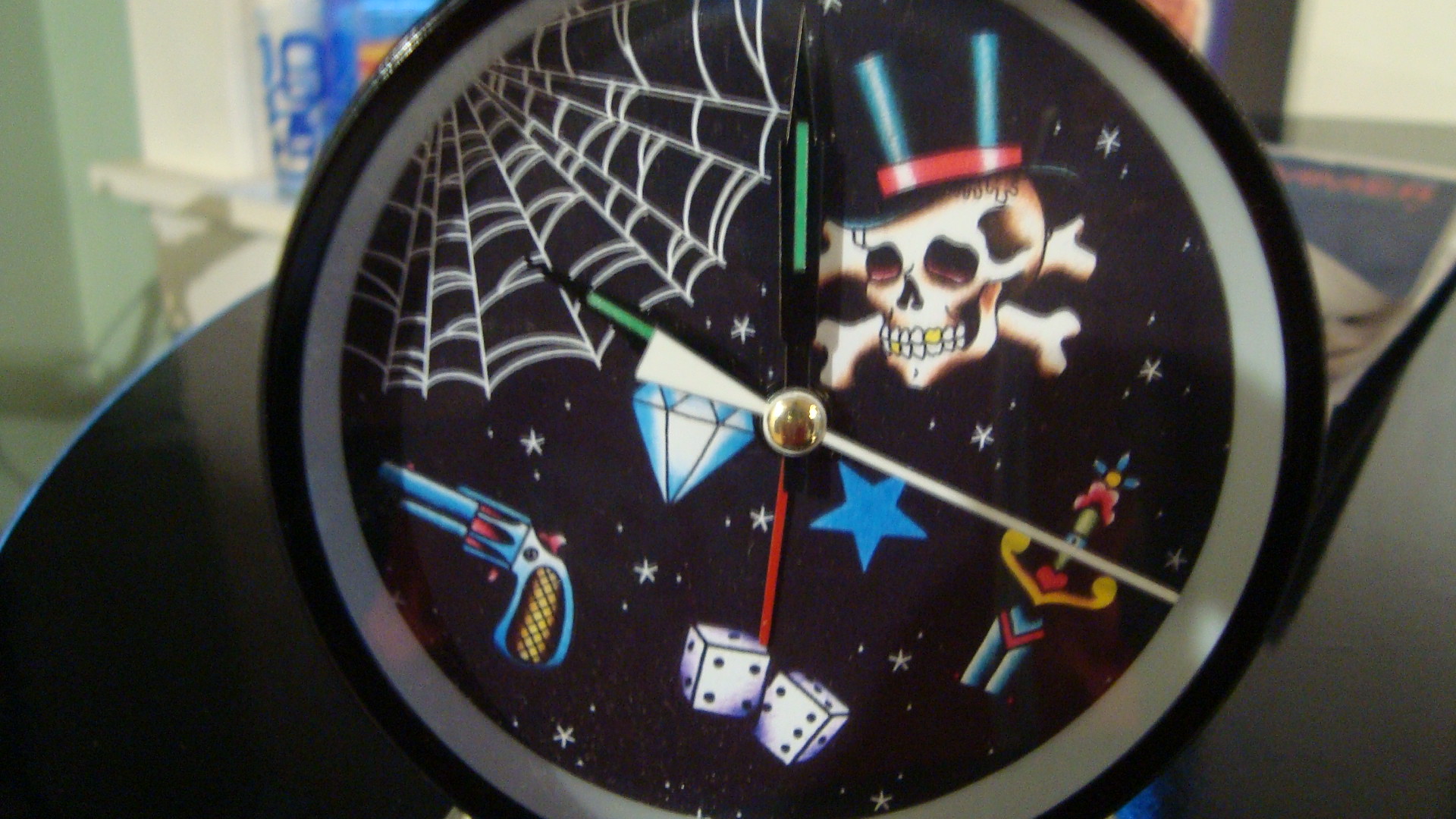A rectangular image showcases a uniquely designed wristwatch, with its longer side oriented horizontally. The watch's face, enveloped in solid black, features various symbols that make it challenging to discern the exact time, though it appears to be approximately 8:55. The hour and minute hands are black with distinctive green stripes, contrasting against a white second hand. The watch face is adorned with an eclectic array of imagery, including a skull and crossbones wearing a top hat, a diamond, a revolver, two dice, a rocket symbol, and a spider web, all set against a backdrop speckled with stars. The watch band, partially visible at the bottom, is black. This intricate and darkly whimsical design gives the watch a striking and mysterious appearance.